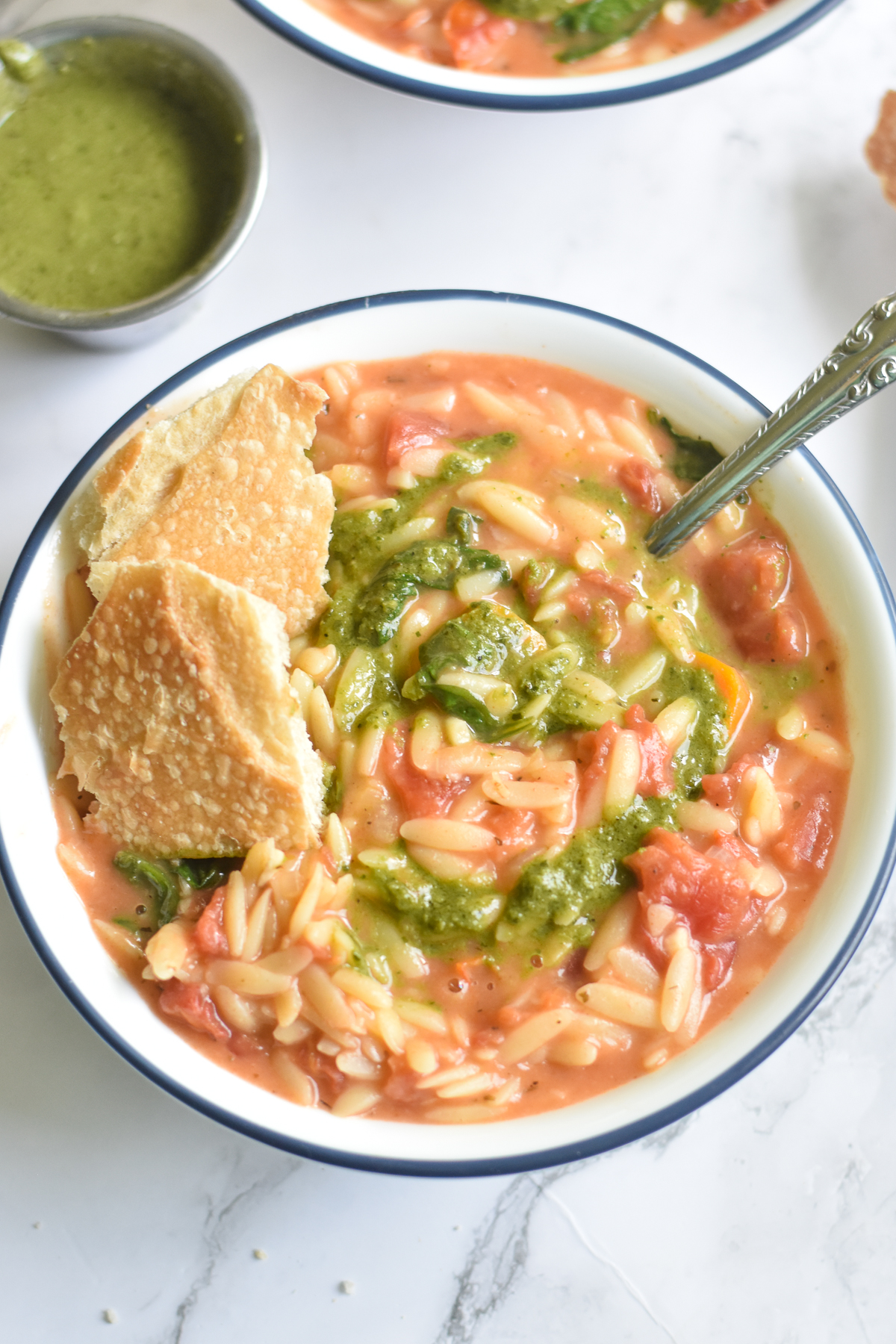The image shows a close-up view of a meal served on a marble countertop. The main focus is a white bowl with a blue rim, filled with a pinkish-red, liquidy soup that appears to contain orzo and tomatoes. A swirl of green pesto decorates the top of the soup. A silver utensil, possibly a spoon with some embossment, is placed inside the bowl, its tip submerged in the soup. To the left of the bowl, there are a couple of chunks of crusty bread. Nearby, there's a small metal cup containing pesto, and just the edge of another similar bowl is visible in the background, indicating a similar presentation. The detail in the image suggests a thoughtfully prepared and visually appealing meal.